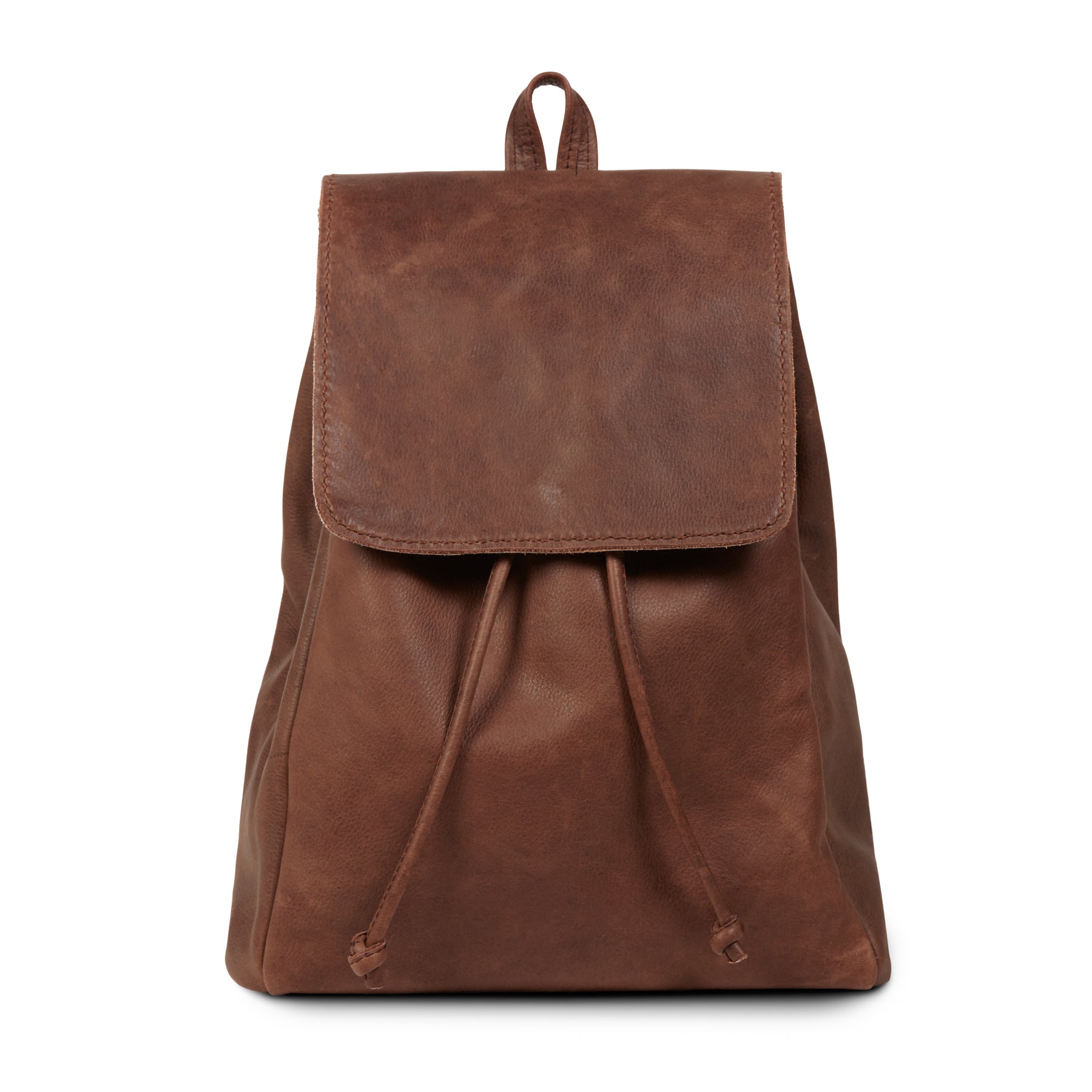A professionally photographed brown leather bag is displayed against a pristine white background. The bag, resembling a backpack or a purse, features meticulous stitching along its top edge and a prominent flap that folds over the front. Two strings, adorned with decorative knots at their ends, dangle from the front of the bag, enhancing its artisanal appeal. The high-quality leather and detailed craftsmanship are clearly visible, making this accessory both functional and stylish.